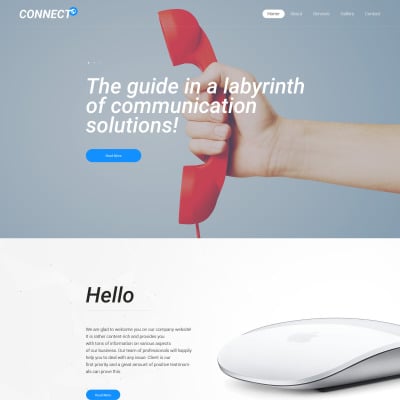This image showcases the homepage of a website called "Connect." The layout is divided into two sections. The upper section features a rectangular area with a grayish-blue background. Superimposed over a slightly grayed-out image of someone holding a red, vintage telephone, there is text that reads, "A guide in a labyrinth of communication solutions." A small blue tab on this section has indistinct text, appearing blurry.

At the top of the webpage, there are four tabs with text that is also too blurred to discern. In the lower section, there's a prominent white square containing an image of an Apple mouse, with the word "hello" clearly visible. The accompanying descriptive text beneath the image is almost entirely unreadable due to blurriness, as are the white words within a small square below this text.